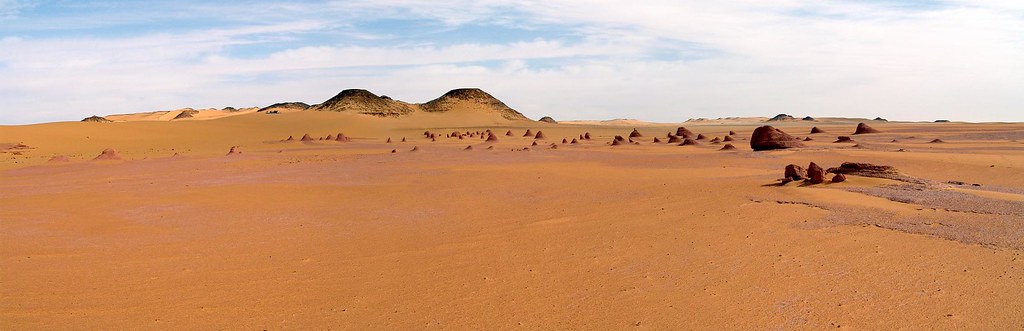The image depicts a wide, horizontal rectangular scene of a desolate desert landscape. The top portion of the image shows a blue sky accented by wispy, semi-evenly strewn white clouds. Below, the landscape is a vast expanse of brown and tan sandy desert, devoid of any vegetation, houses, or identifiable markings. In the foreground, there is reddish-brown sand, and scattered throughout the middle of the image are rounded, rock-like formations, resembling clay and sandy boulders. Dominating the background are two large, black-tipped hills or old volcanoes, positioned slightly left of center. The expansive, barren desert extends uninterrupted, emphasizing the stark, lifeless beauty of the scene.